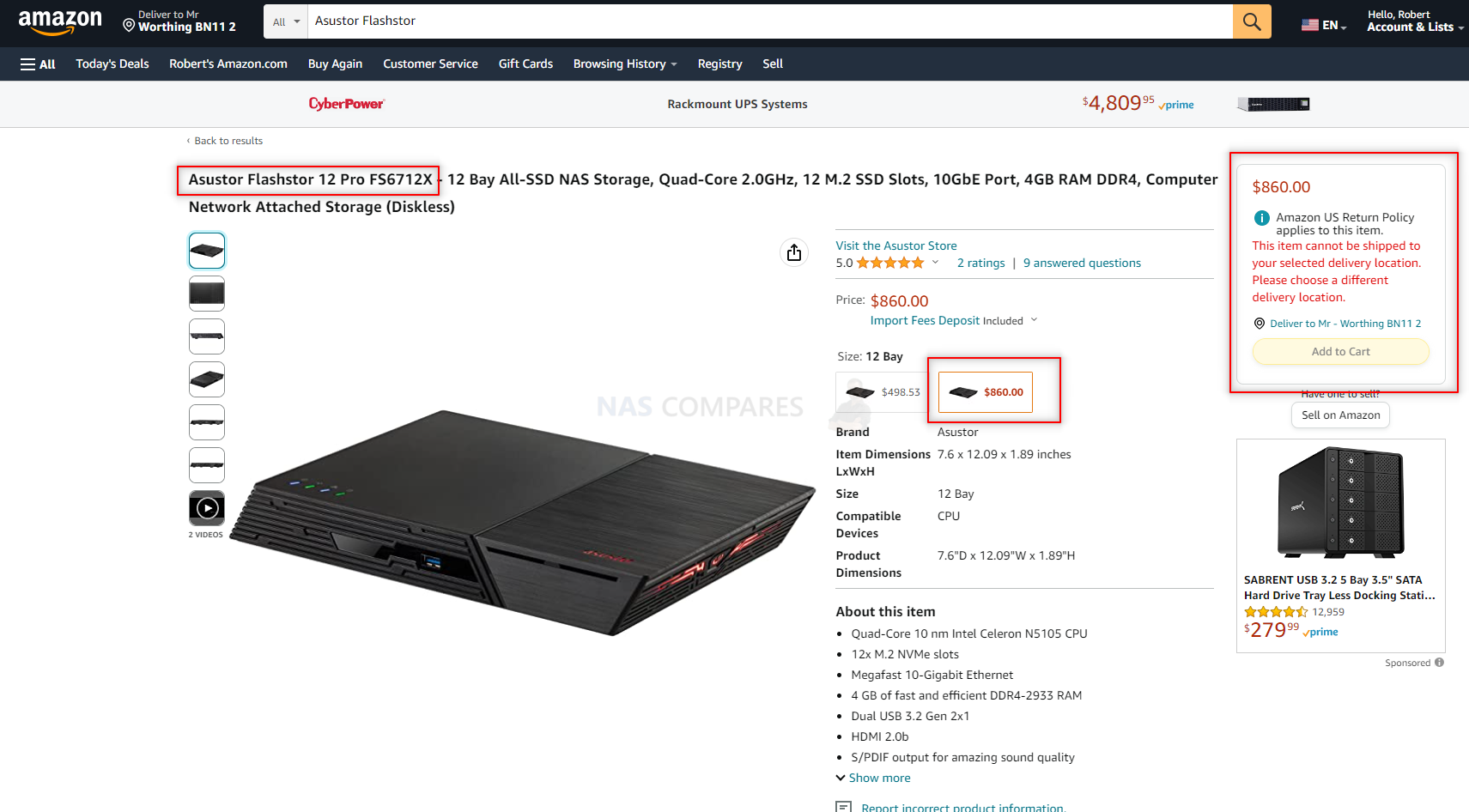**Detailed Caption of an Amazon Product Page**

The screenshot captures an Amazon webpage. In the top-left corner, the familiar Amazon logo is present, adjacent to the delivery destination information. To the right, there is a search bar, and further along, it says "Hello, Robert" with links to his account and lists. Below this header, there is a navigation bar featuring various tabs like "Today's Deals" and "Browsing History."

The main section of the page showcases what appears to be a hard drive, specifically a network attached storage device. The product image depicts a sleek, black, square box with angled sides. Four lit circles adorn the left side of the box, though their exact nature is indistinct. The right side displays what is likely the brand name in red text. The front and left sides feature jagged slots that suggest design intricacy and utility.

To the left of the main image, three smaller images show the product from different angles, accompanied by two video thumbnails. 

At the top of the product description, the name is prominently displayed within a red rectangular box: "ASUSTOR Flashstor 12 Pro FS6712X". The description continues, highlighting key specifications such as its 12-bay storage capacity, quad-core 2.0 GHz processor, 4GB RAM, and diskless network attached storage (NAS) capabilities.

On the right side, the price is listed at $860.00, shown alongside a lower-priced option at $498.53. The product has a perfect 5.0 rating based on two reviews and includes nine answered questions. Additionally, there is a link to visit the ASUSTOR store.

Further details list product dimensions and features like gigabit Ethernet and HDMI ports, with additional information accessible by clicking "Show More." 

A highlighted box in the upper-right corner alerts the user that the "Amazon US return policy applies," but it also indicates that the item cannot be shipped to the selected location, suggesting an alternative delivery address needs to be chosen.